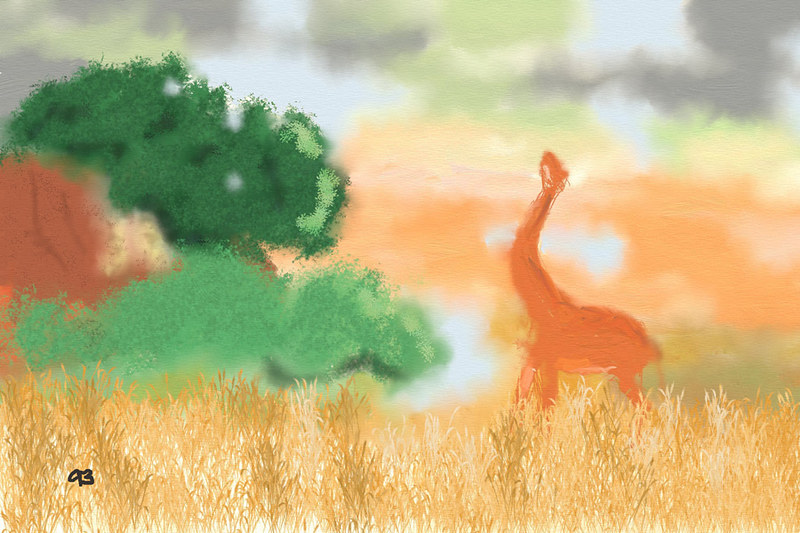The painting depicted in the image portrays a serene nature scene, capturing the essence of a dry, grassy landscape. At the bottom of the painting, hues of yellow and beige dominate, effectively representing the parched grass typical of a sun-soaked savanna. In the background, towards the left side of the canvas, a spectrum of green shades intersperses with the yellow, likely simulating a pocket of trees or dense foliage offering a burst of life amidst the aridity. 

On the right side, an intriguing and whimsical orange figure commands attention. This creature, possibly inspired by either a giraffe or a dinosaur, is depicted in a simplistic, almost abstract manner, characterized by its long neck extended skyward. Despite its lack of intricate detailing, the orange silhouette injects a sense of curiosity and imagination into the scene. The painting is devoid of any text, allowing the viewer to immerse fully in the visual narrative crafted through color and form.